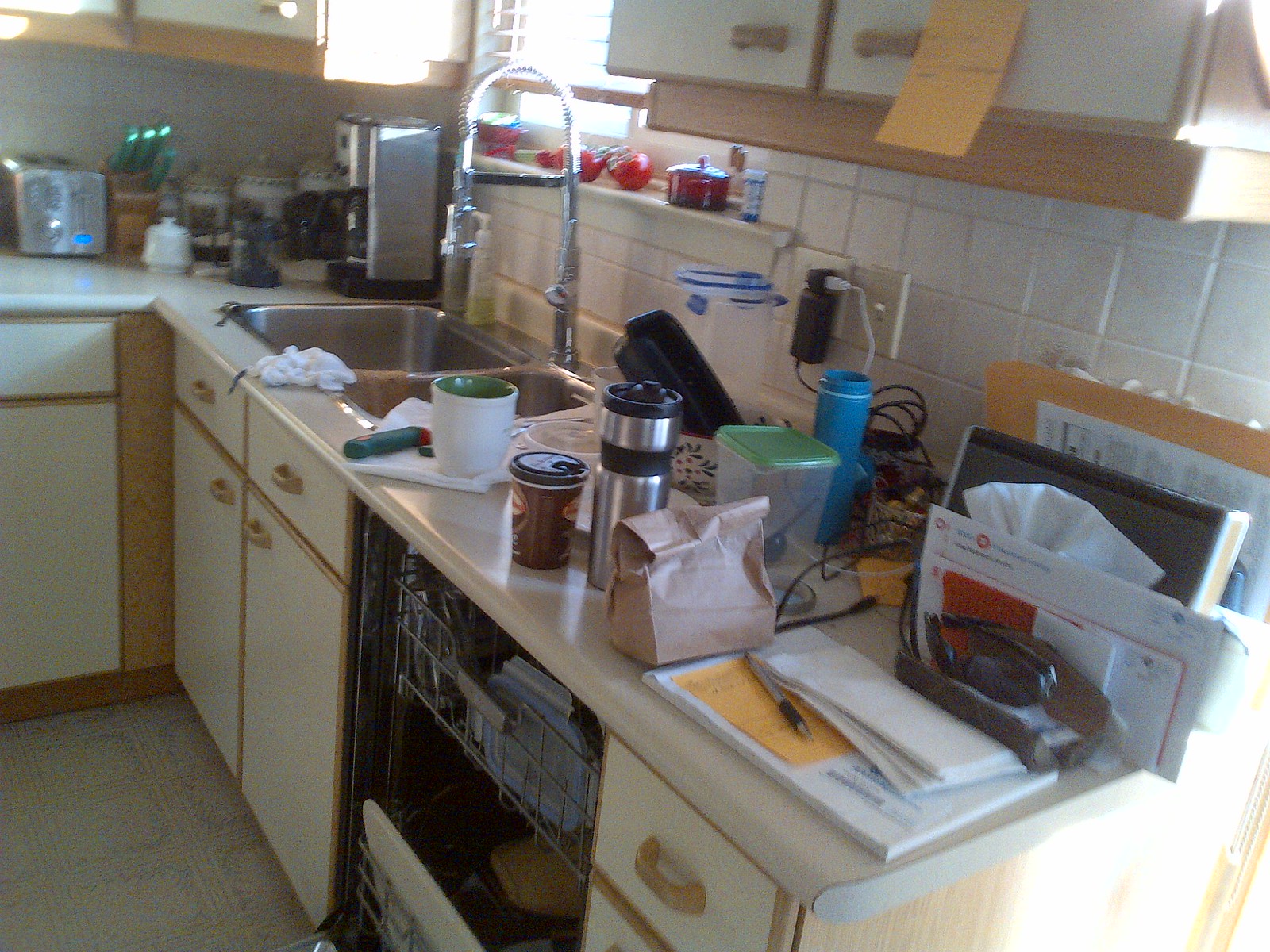The image captures a detailed view of a well-used kitchen area. The floor is adorned with light-colored tiles in a beige and blue pattern. The white cabinets feature a natural wood trim and matching light wood handles, accentuating their clean yet rustic aesthetic. A pristine white countertop runs atop these cabinets, hosting a double bowl sink at its center. To the far right under the countertop, an open dishwasher is visible, indicating recent use.

The countertop itself is cluttered with various items, evoking a sense of daily life and activity. Food storage containers, a thermos, a paper bag, a ceramic coffee cup, and a to-go cup from a restaurant are strewn across its surface. Above the sink, a small shelf holds some ripe tomatoes, adding a touch of color and freshness to the scene. The walls around the shelf and sink are covered with white ceramic tiles, contributing to the kitchen's clean and classic look. 

To the far right of the countertop, a mail holder is affixed to the wall, designed to organize mail and other paperwork. The image contains no text, allowing the viewer to focus solely on the intricacies and lived-in quality of the kitchen space.